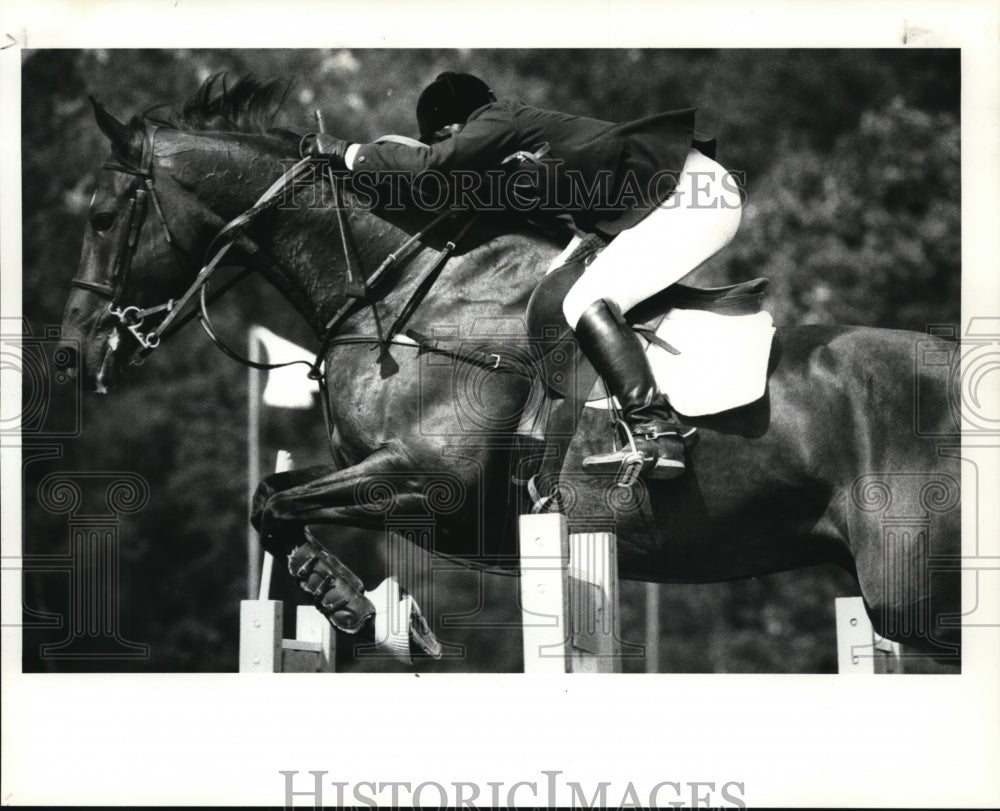This black and white photograph captures a dramatic moment during an equestrian event, featuring a jockey and their horse in mid-jump over a hurdle. The horse is frozen in motion, with its front legs elevated, hooves airborne as it faces towards the right. Unfortunately, the back legs are not visible in the frame. The determined jockey, slightly elevated off the saddle, is wearing white pants, black boots, a dark jacket, and a dark hat, with a riding crop grasped in the left hand; the right hand is out of view. The horse appears to be a solid color, possibly chestnut or black, though the monochromatic nature of the image obscures this detail. The photograph has watermarks that read "Historic Images" at both the top and bottom, and additional markings resembling sketch cameras are subtly visible in the background. Hints of trees can also be seen, indicating that the event is taking place outdoors.